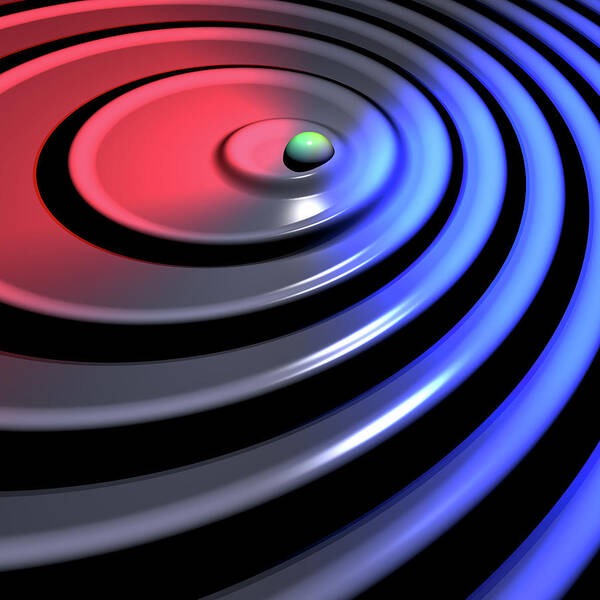This square image, about four to five inches in height and width, presents a complex, multi-layered circular design. At the center of the image, there is an irregularly shaped green dot, shaded gray at the center and black at the bottom, situated within a depressed circular ring. This central ring is nested within a series of progressively larger rings, each defined by a unique coloration and depth, enhancing the three-dimensional effect. Starting from the top center, each ring expands outward, with the upper left-hand corner of the rings illuminated in red light. Transitioning to the right, both the upper and lower right-hand corners display rings accented in light blue. The bottom and bottom left regions feature gray rings, each outlined starkly in black to delineate the depth variations.

Towards the bottom right corner, the sequence of alternating colors becomes more intricate, with black and blue lines repeating. The central portion of the larger rings exhibits shades of pink, particularly towards the top left corner and extending through two outer loops. The design on the right side shifts more towards blue. Another ring near the center lacks the black outline, maintaining a pure form that contrasts with the rest. Overall, the image resembles a set of concentric loops, reminiscent of heated stovetop elements or sound waves, although it is purely abstract in nature. The design does not feature any text, maintaining its focus on the intricate, visually captivating pattern.